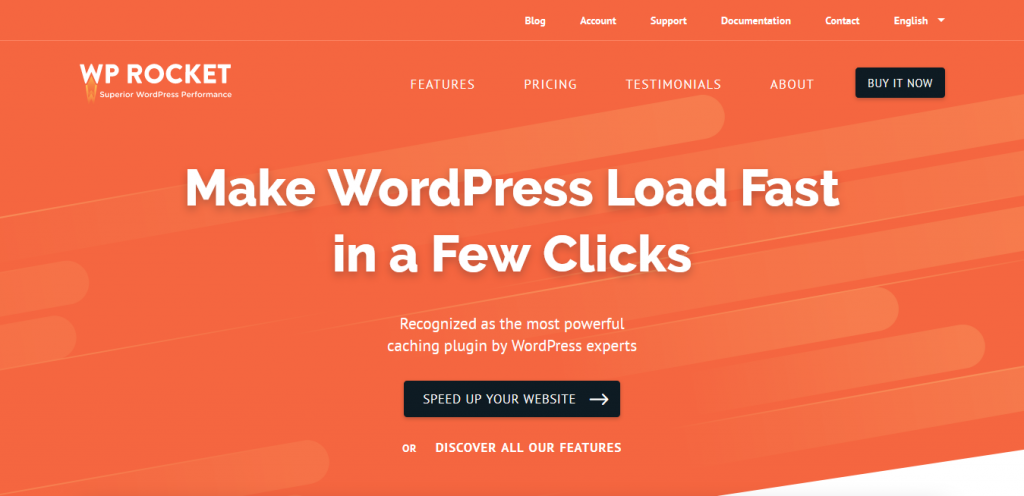This image showcases a vibrant website with a reddish-orange background that features transparent, elongated, rounded-off oval ends and random geometric strips as a graphic design element. The primary text throughout the site is white, creating a sharp contrast against the background. The top menu includes the following items separated by small dividers: Blog, Account, Support, Documentation, Contact, and a dropdown menu for language selection, defaulted to English.

On the left side of the page is the WP Rocket logo followed by the tagline "Superior WordPress Performance" in a bold, all-caps, sans serif font resembling Helvetica. White text below the logo provides navigation to Features, Pricing, Testimonials, and About, which are positioned next to a prominent black "Buy It Now" button located in the upper right corner. 

The central focus of the page is a large, attention-grabbing headline that reads "Make WordPress Load Fast in a Few Clicks." Directly below this headline is a brief description in smaller text, stating "Recognized as the most powerful caching plug-in by WordPress experts." Additionally, there's another black button at the bottom middle of the page that reads "Speed Up Your Website," accompanied by a right-pointing arrow.

Beneath this call-to-action button, smaller, all-caps text offers an alternative action: "OR, Discover All Our Features."